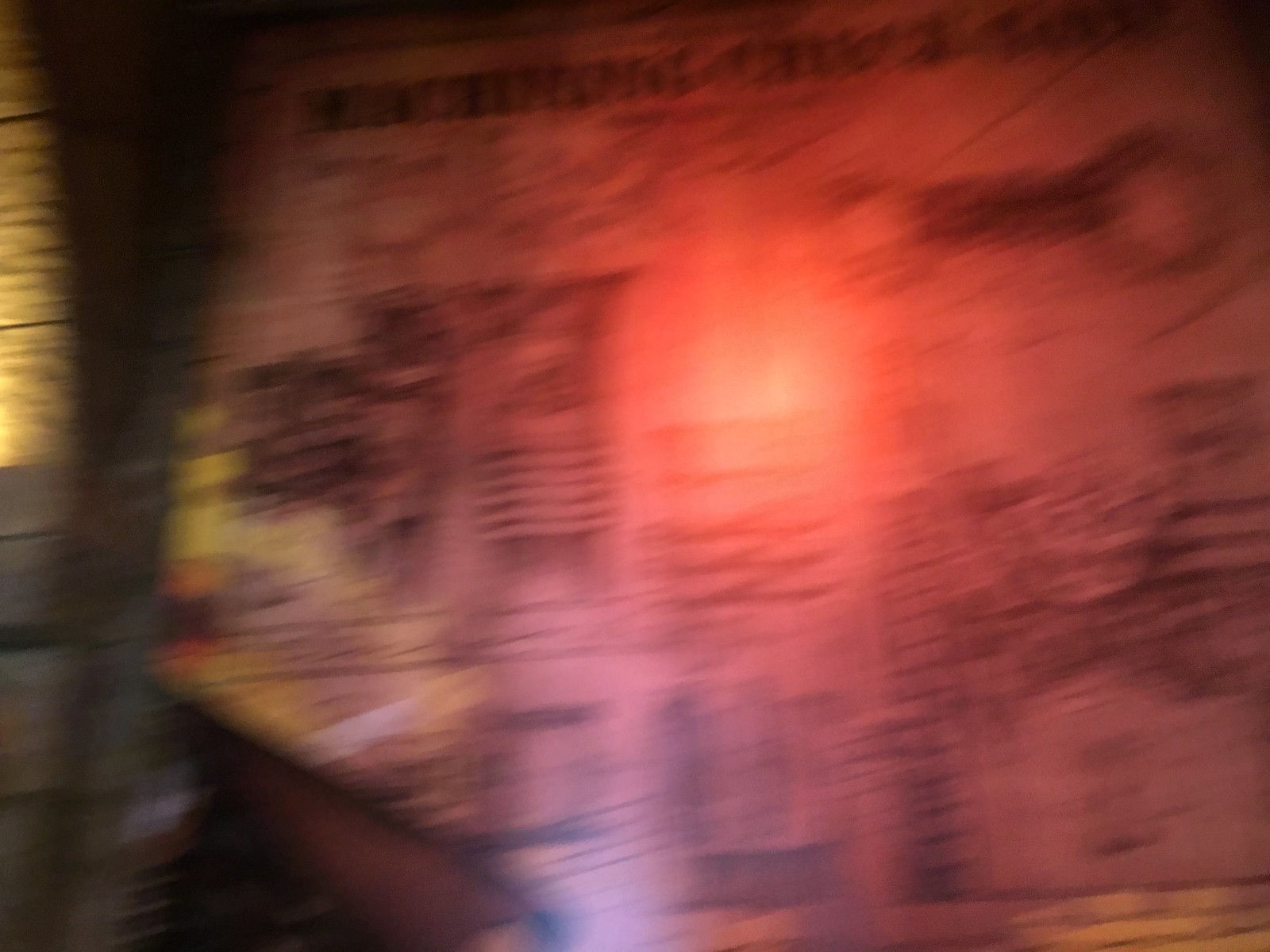This blurred photograph captures a graffiti-like mural on a wall, reminiscent of a moth's shape. A red light's reflection casts an eerie glow on the mural, adding an otherworldly atmosphere. The top of the image features black text, while beneath it, a series of indistinct dark graphics are visible, their details lost to heavy blurring. On the left side, a portion of a tan wall is discernible, with an overlay of white shadow-like forms. A yellow light and scattered black lines contribute to the chaotic scene. The moth-shaped mural itself is accentuated with patches of yellow, orange, and streaks of black, adding vibrant yet dark tones to the artwork.